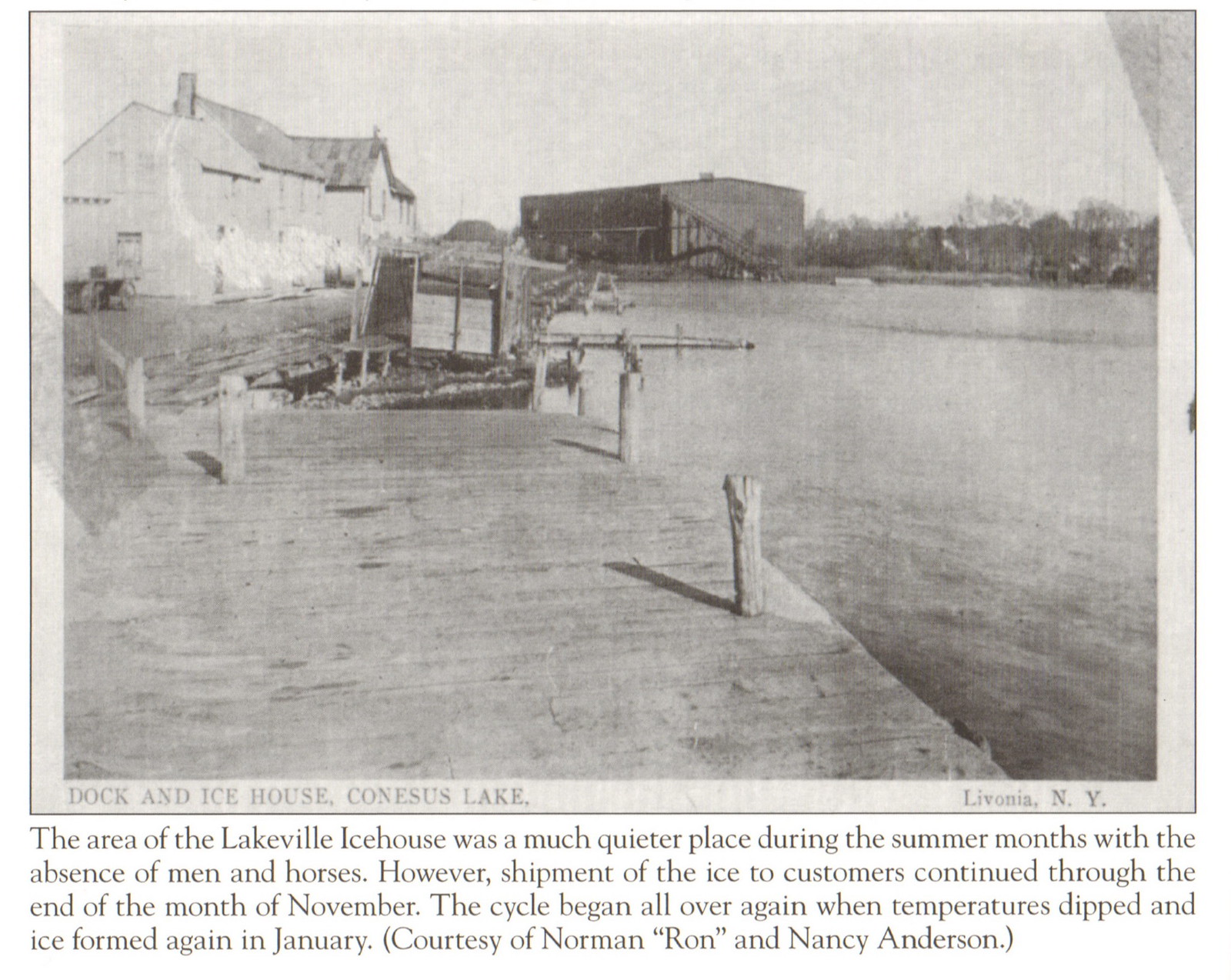A black-and-white photograph captures a serene lake scene at Canisius Lake in Livonia, New York. Central to the image are two buildings, identified as the Dock and Ice House, situated to the left of the lake, with a wooden dock extending into the water. Detailed text beneath the photo reads: "The area of the Lakeville Ice House was a much quieter place during the summer months with the absence of men and horses. However, shipment of the ice to customers continued through the end of November. The cycle recommenced when temperatures dipped and ice formed again in January. Courtesy of Norman, Ron and Nancy Anderson."